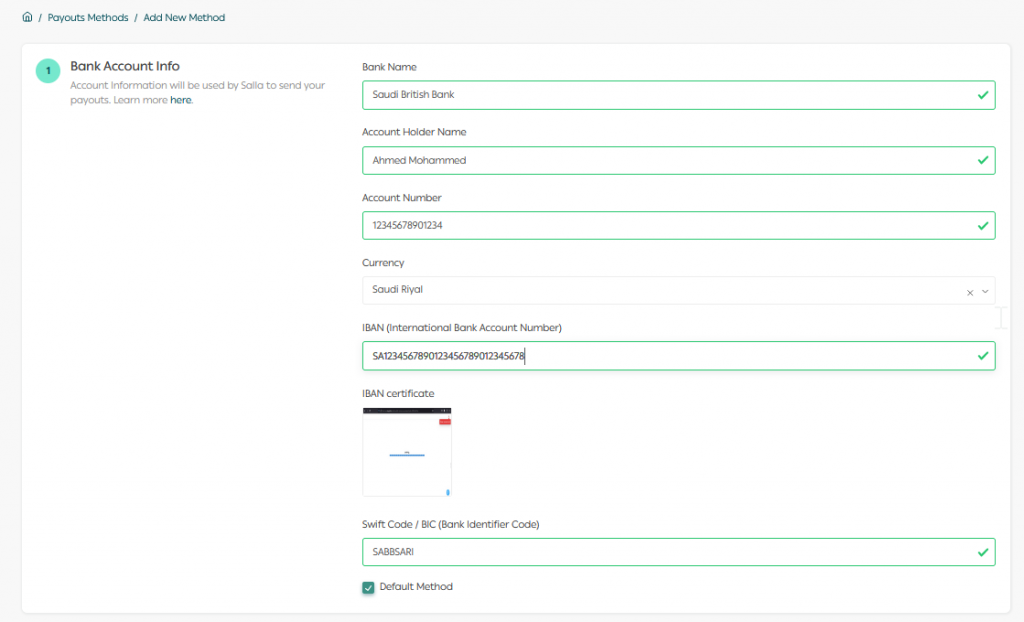This rectangular image features a light gray border, which is very thin on the bottom and right sides, slightly thicker on the left, and distinctly thicker at the top. At the top of the image, there is green text which reads "Payout Methods" and "Add New Method," with a small home icon to the far left. 

The main content of the image is housed within a white section labeled "Bank Account Info." A green circle with the number "1" is adjacent to the text that says, "Account information will be used by Salia to send your payouts. Learn more here," with the word "here" highlighted in blue, indicating a hyperlink.

Further to the right, the image displays detailed bank information: 

- **Bank Name**: Saudi British Bank
- **Account Holder Name**: Ahmad Muhammad
- **Account Number**: [Number present]
- **Currency**: Saudi Riyal
- **IBAN**: [IBAN Number present]
- **IBAN Certificate**: [IBAN Certificate present]
- **SWIFT Code**: [SWIFT Code present]
- **Default Method**

Each of these sections is highlighted in green and contains check marks, except for the "Currency" section. 

This meticulous layout ensures clarity and organization, making it easy to review the bank account details and payout methods.